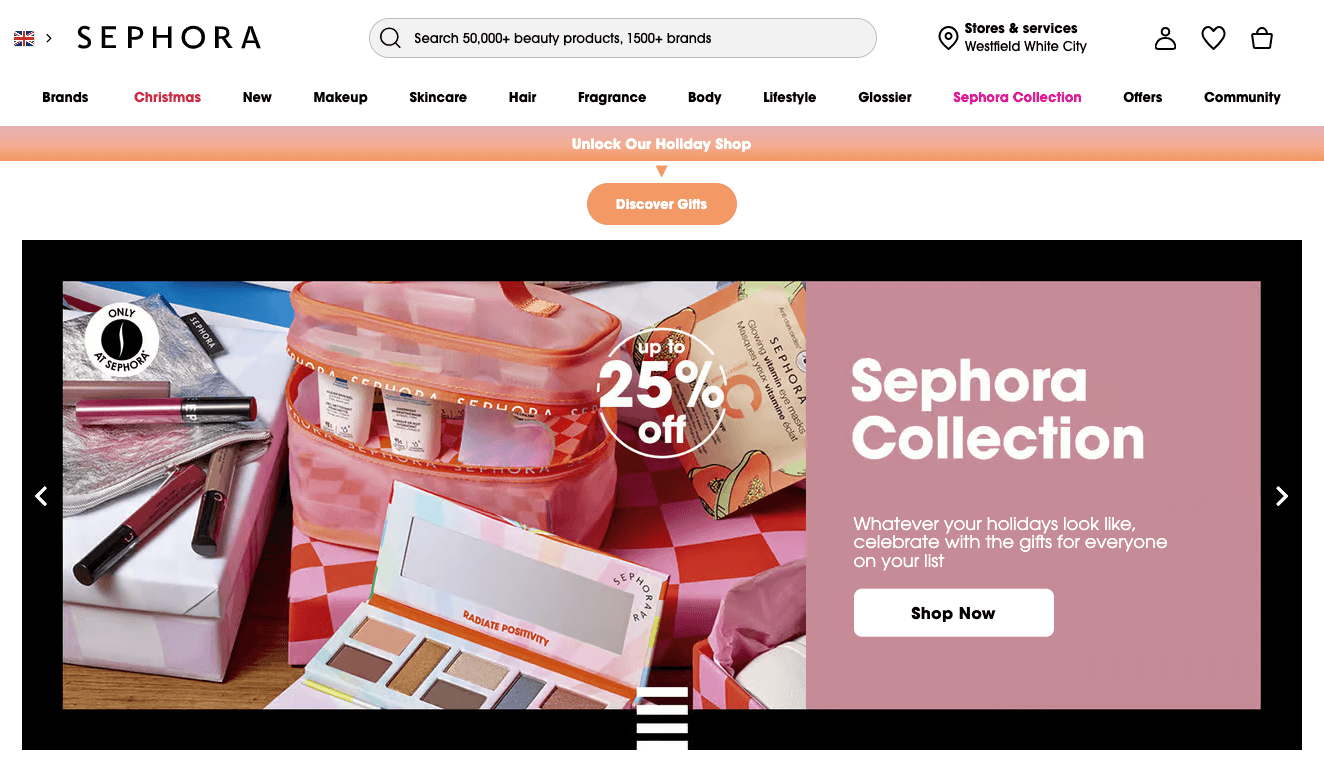The horizontally rectangular image is a screenshot of the Sephora website. In the top left corner, the "Sephora" logo is prominently displayed. To its right is a search field containing the text, "Search 50,000+ beauty products, 1,500+ brands." Moving further right, there are links for "Stores & Services" accompanied by a location icon, indicating the locale as Westfield White City. Additionally, the profile, favorites, and shopping cart icons are aligned to the right.

Just below this, a horizontal menu bar showcases various categories labeled as: Brands, Christmas, New, Makeup, Skincare, Hair, Fragrance, Body, Lifestyle, Glossier, Sephora Collection, Offers, and Community. All these categories are rendered in black text, except for "Christmas" highlighted in red and "Sephora Collection" in pink.

Beneath this menu, a promotional banner reads "Unlock Our Holiday Shop," accompanied by a "Discover Gifts" button. Below this banner, a horizontally rectangular image spans the width of the frame, displaying a makeup case filled with various makeup items. Overlaid text indicates a discount of "Up to 25% off." To the right of this image, a section titled "Sephora Collection" presents the tagline, "Whatever your holidays look like, celebrate with the gifts for everyone on your list," followed by a "Shop Now" button.